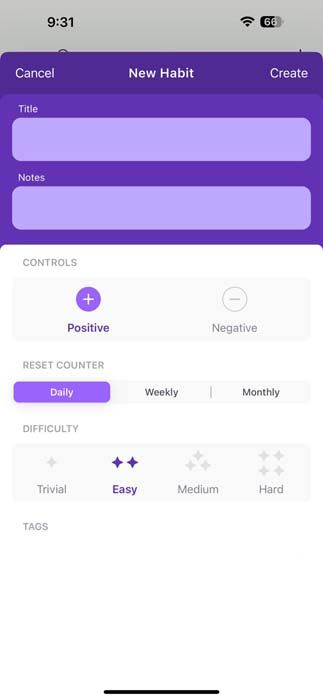This image showcases a smartphone application designed for habit tracking. The app interface is mainly set against a white background, with the top third featuring a dark blue header. Within this header, there is a mock-up of an older iPhone, complete with typical phone interface elements. At the top of the app, there are options to either "Cancel" or "Create" a new habit. 

A text box allows users to enter a title for the new habit, and there is an option to add notes. Below this, still on the white background with royal blue accent colors, users can choose to mark the habit as positive or negative, with the positive option currently selected.

Further down, the app offers settings to reset the habit counter daily, weekly, or monthly. The difficulty level is displayed in gray with "Easy" chosen, which is part of a scale ranging from "Trivial" to "Hard." Each difficulty level is associated with star ratings: one star for Trivial, two stars for Easy (which is highlighted), three stars for Medium, and four stars for Hard. The difficulty level selector also appears in gray.

Tags can be added to the habit, providing more customization. At the bottom of the screen, the distinctive iPhone home bar is visible, indicating that this interface is a mock-up from when the home bar feature was initially introduced on older iPhones.